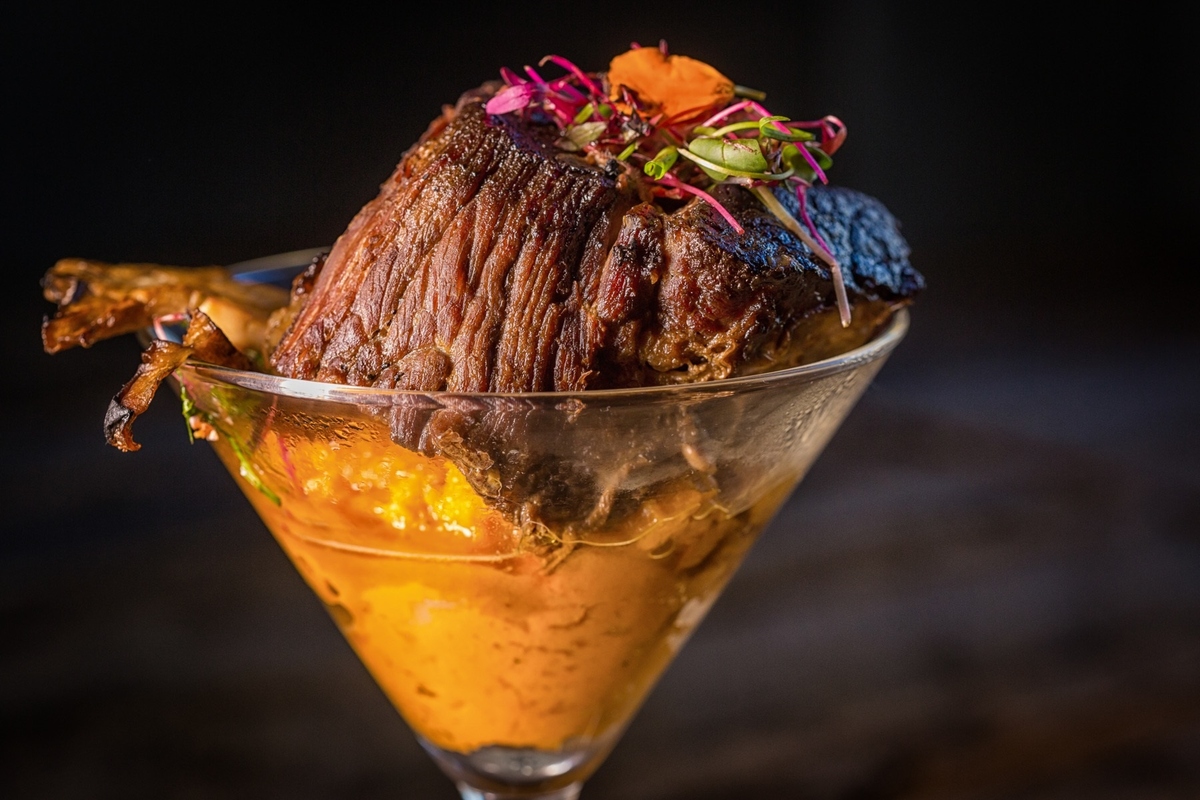This close-up photograph showcases the top of a martini glass filled with an intricate and unsettling culinary creation. The glass, only visible from the top, is seated against a dark, blurred background that heightens the focus on its unusual contents. Inside, a vivid orange liquid fills roughly three-quarters of the glass, reminiscent of an orange slushy or muddle. Perched atop this bright base is a large, thick cut of blackened steak, partially charred and garnished with an array of decorative edibles, possibly including thyme and beet-colored greens. Adding to the bizarre ensemble is what looks like a collection of colorful insects, including an orange spider, a green grasshopper, and a blue insect, all arranged on what seems to be a scoop of chocolate ice cream resting on the steak. Additionally, a shrimp or crab leg protrudes from the left side of the glass, and an amphibian-like creature, resembling a frog, lingers on the rim with its head and forearms hanging out. The overall composition is visually striking yet grotesque, creating a chaotic and unappetizing display.